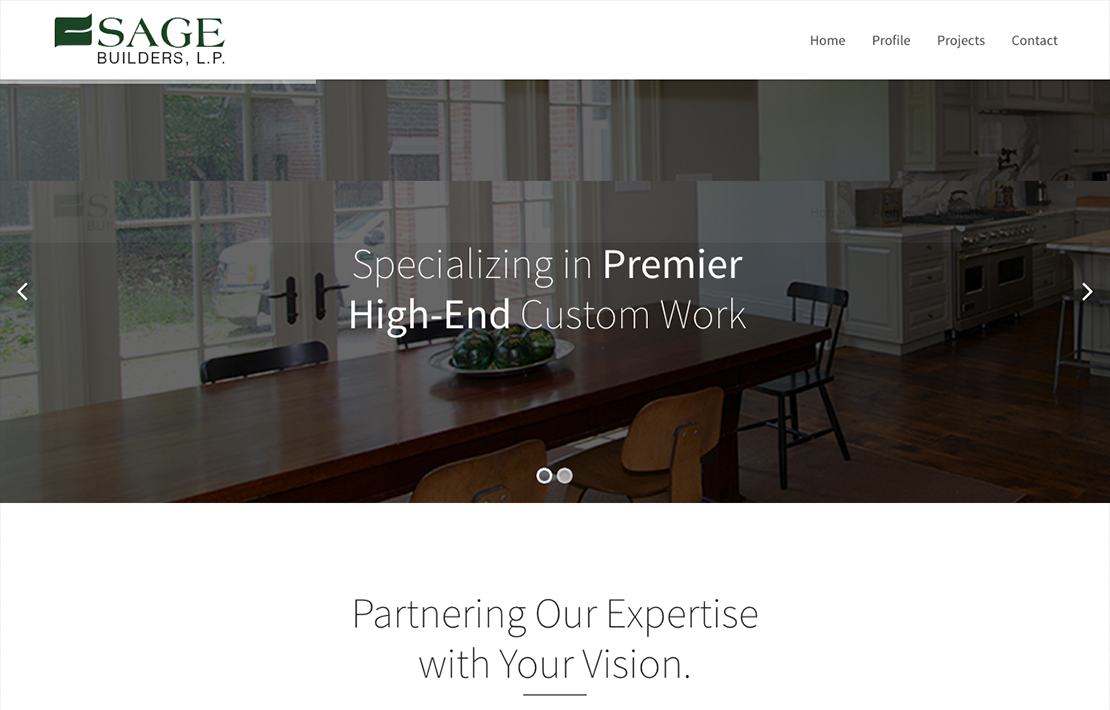This image captures the main page of the 'Sage Builders, LP' website. At the top, the company logo features the word 'Sage' in a distinctive mossy green font, while 'Builders, LP' is displayed below it in black. Prominently placed is the company slogan, "Partnering our expertise with your vision," also in black font. The bottom portion of the page showcases a slideshow, currently displaying an inviting kitchen setting within a home. This cozy kitchen features a dark wood table, surrounded by an eclectic mix of mismatched chairs. French doors provide an airy backdrop to the open kitchen floor plan. The webpage emphasizes the company's expertise with the phrase, "Specializing in premier high-end custom work." Navigation tabs at the top of the page include 'Home,' 'Profile,' 'Projects,' and 'Contact,' allowing users to explore further.